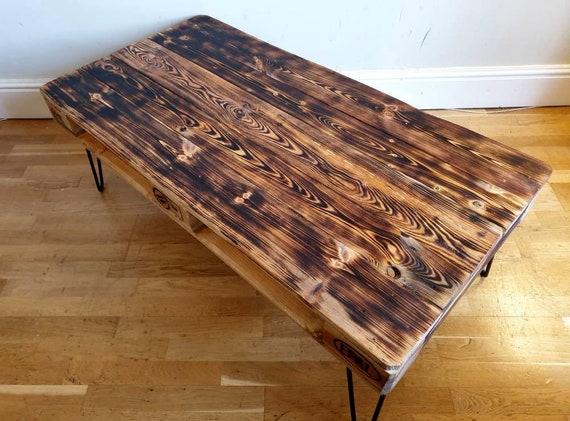The image portrays a rectangular, homemade wooden bench wider than it is tall, positioned diagonally from the top left to the bottom right corner. The bench, constructed from light-colored wood with black, darkened markings that give it a marbled or stained appearance, rests on thin, black metal legs shaped in a V formation. This piece, which could also be interpreted as a small table due to its wide surface, sits on a traditional hardwood floor composed of lighter brown, rectangular planks. The background features a pristine white wall with an unobtrusive white baseboard running along its bottom. The image captures only the lower portion of the wall, providing a minimalist aesthetic. Notably, the wood's natural patterns and grooves stand out, and a small, rectangular notch with an illegible drawing and logo is visible on the side of the bench. There are no other objects, decorations, or prominent features in the room, making the bench the focal point of the scene.